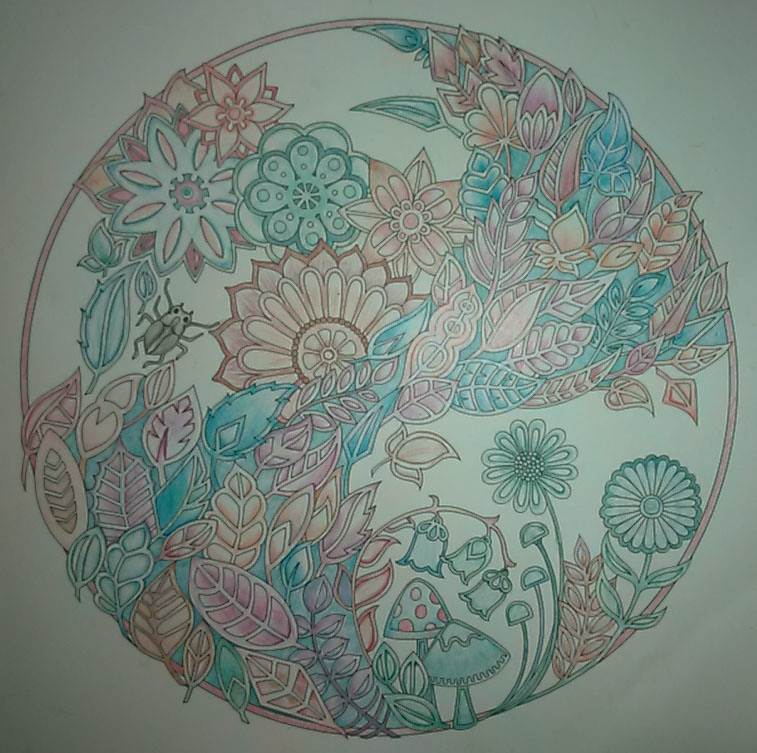This meticulously colored photograph captures an exquisite drawing, possibly an original piece or a detailed coloring book illustration. The image is filled with vibrant shades of orange, pink, blue, and green, all skillfully blended using colored pencils. At its center, a lush scene unfolds within a circular frame, bordered by a rich reddish hue.

Within the circle, intricate depictions of greenery and foliage stand out, accompanied by a diverse array of flowers. A small black beetle is discreetly placed in the left section, adding a touch of natural realism. The background is adorned with various designs, including suns, floral patterns, and additional decorative elements.

Adding a whimsical touch, several mushrooms, including charming little toadstools, are scattered throughout the scene. Toward the bottom, dainty bell-shaped flowers contribute to the overall enchanting atmosphere of the illustration. This artwork is a testament to meticulous craftsmanship and vibrant creativity.